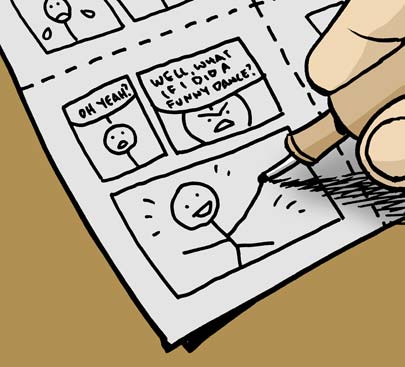The image illustrates a comic strip being actively drawn by an artist. The comic is rendered on a white sheet of paper positioned on a light brown table. The artist's hand is visible, specifically the forefinger and thumb, which are grasping a fine-point pen with a light tan body and a black tip. The comic itself features a series of stick figures, each exhibiting distinct facial expressions and thought bubbles. In the upper left corner, a stick figure with a sad face, complete with two tears, can be observed. In the lower left corner, another stick figure exclaims, "Oh yeah?" followed by a third stick figure with a scowling face saying, "What if I did a funny dance?". The final cell depicts the stick figure with a broad smile and limbs spread out, appearing to dance. Overall, this comic strip captures a sequence of emotional reactions and humorous actions conveyed through minimalist yet expressive stick figure art.